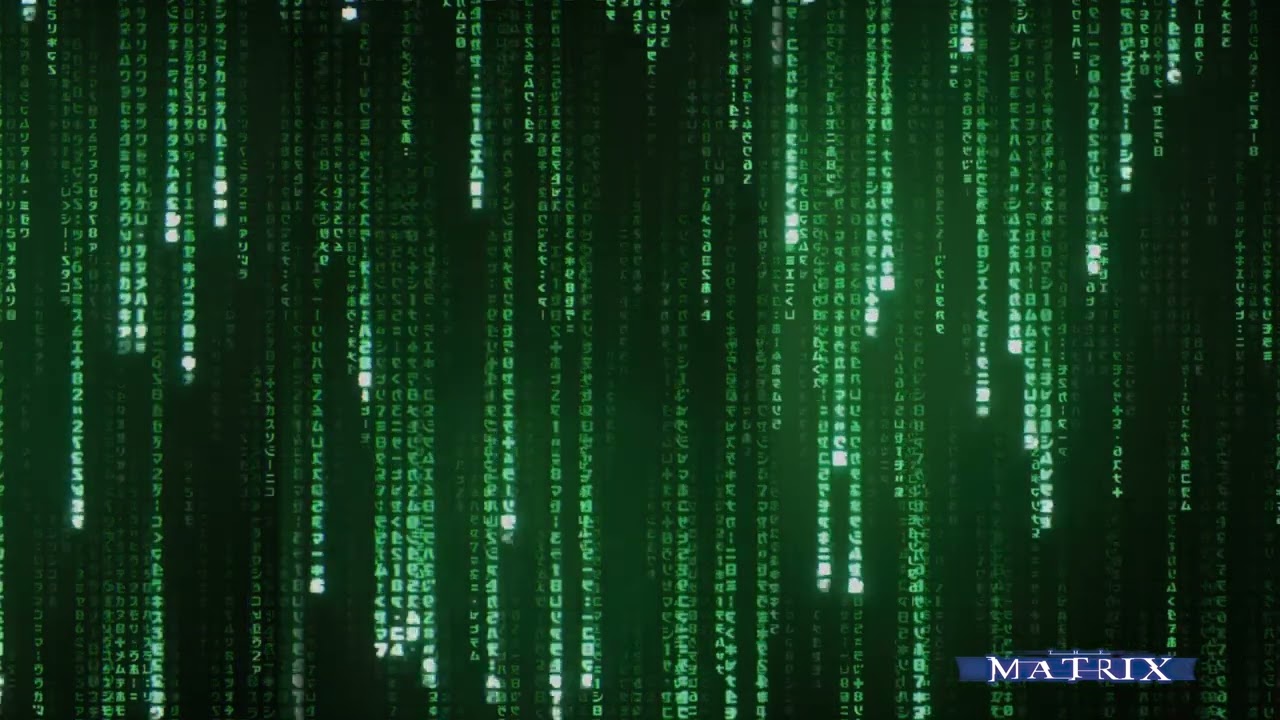This image depicts the iconic falling green text from the movie *The Matrix*, showcasing vertical strands of neon-green characters cascading down a pitch-black background, reminiscent of rainfall. The characters, a mix of nondescript hieroglyphics and vaguely Asian symbols, illuminate variably, growing brighter at the bottom of each strand. Across the entire image, these luminous green text streams of different lengths extend from the left side, growing longer towards the middle, and then shortening again towards the right. In the bottom right-hand corner, the text "The Matrix" is prominently displayed in a distinct, etched-font style, adding a recognizable touch to the digitally immersive scene.